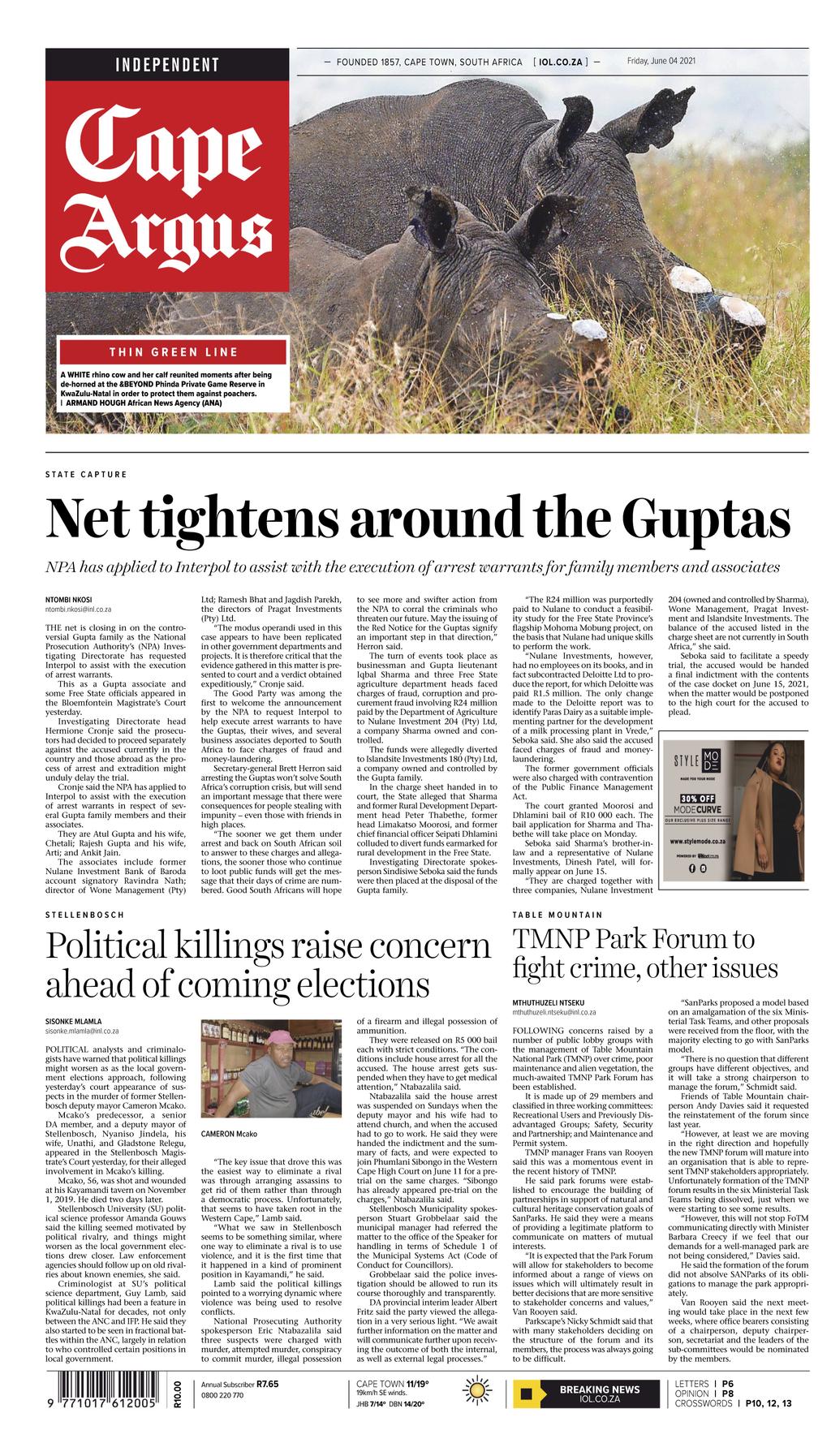The image appears to be a screenshot or photograph of a website or a newspaper front page, specifically from the "Independent Cape Argus." The heading "Founded Cape Town, South Africa" is prominently displayed at the top. The main image features two rhinoceroses with their horns visibly sawed off, leaving one to ponder their fate.

The newspaper's name, "Cape Argus," is distinctively highlighted in an artsy font housed within a red box. The headline article on this front page, "Net Titans Around the Guptas," is printed in the largest font and draws immediate attention.

Additionally, there is an advertisement featuring a woman dressed in a beige jacket. Two other articles are also visible: "Political Killings Raise Concerns Ahead of Coming Elections," and "TMNP Park Forum to Fight Crime and Other Issues." These articles are fully legible, offering insights into political and social issues in the region.